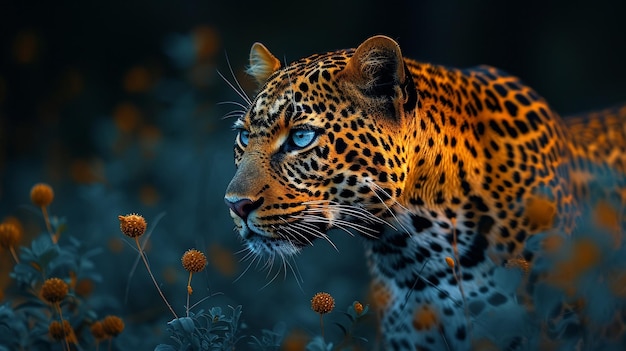The image features a digitally enhanced, color-saturated depiction of a large feline, most likely a cheetah due to its distinctive black spots on its vibrant orange fur. The cheetah is positioned centrally in a horizontal landscape orientation, facing left. Its large blue eyes and white-furred chin and belly, speckled with black spots, are sharply in focus, providing a striking contrast to the blurred, dark background. Surrounding the cheetah are clusters of orange pom-pom flowers that blend harmoniously with the animal's fur. These flowers appear intermittently in both the foreground, notably on the bottom left corner, and in the background, adding to the layered depth of the image. Subtle digital enhancements, including a slight vignette and luminescent effects, further highlight the cheetah's vibrant coloration and detailed features, emphasizing its surreal and almost painterly appearance.